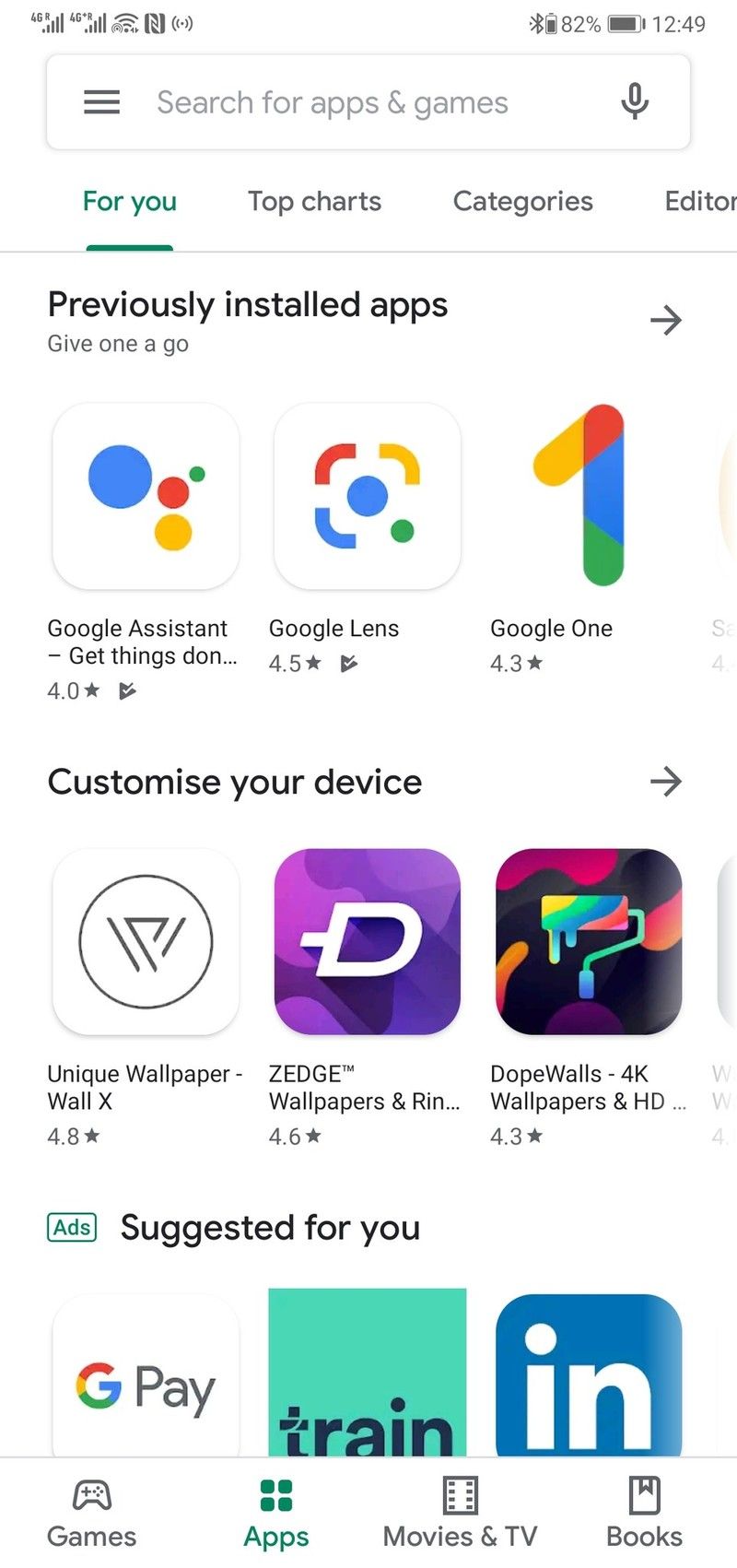Here's a cleaned-up and detailed caption for the image:

---

This image is a screenshot from the Google Play application, showcasing a user interface from an older version of the app in light mode. 

**Top Bar:**
- **Top Right Corner:** 
  - Time: 12:49 PM
  - Battery Status: 82% charged
  - Bluetooth Icon
- **Top Left Corner:** 
  - Signal Strength Indicators: 
    - LTE signal strength
    - Wi-Fi signal strength

**Top Section:**
- **Search Bar:** Positioned below the status indicators, the search bar is labeled "Search for apps and games."
- **Navigation Tabs:** Located horizontally below the search bar, the tabs include:
  - For You
  - Top Charts
  - Categories
  - Editor's Picks

**Main Body:**
- **App Listings:** The main section displays a variety of app icons with their names and star ratings. The apps shown are:
  - Google Assistant
  - Google Lens
  - Google One
  - Google Play
  - LinkedIn
  - Zedge
  - Dope Walls
  - Unique Wallpaper, WallX

**Bottom Navigation Bar:**
- **Menu Options:** At the very bottom, a small bar menu lists four options:
  - Games
  - Apps
  - Movies & TV
  - Books

**Additional Details:**
- The interface is set against a light background, indicating the app is in light mode.

---

This caption provides a clear and detailed description of the screenshot, outlining the various elements and sections visible in the image.